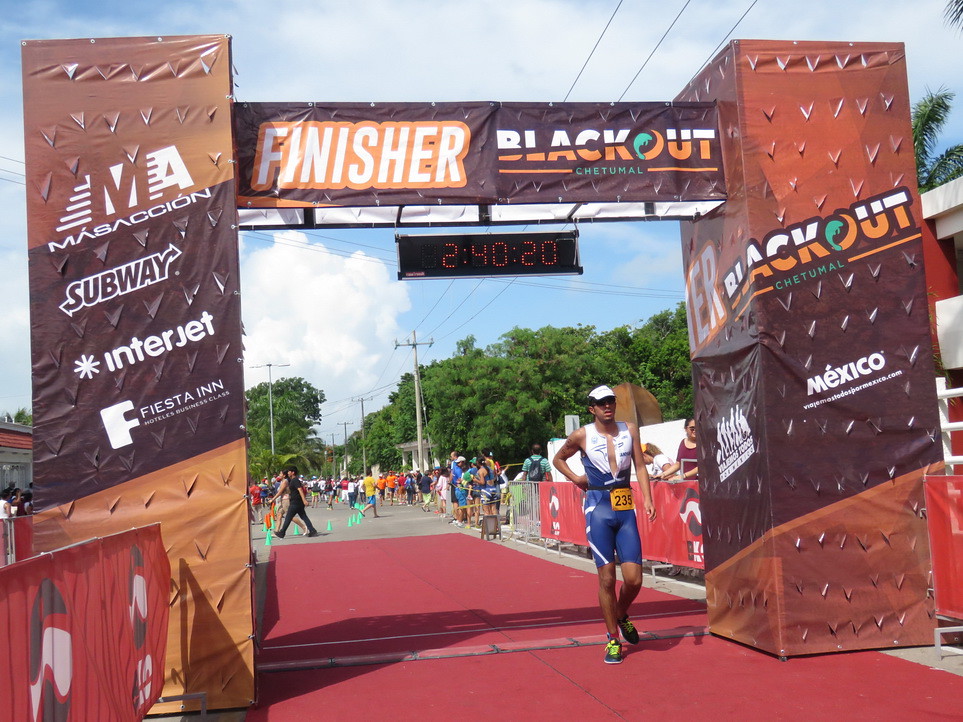The image depicts the finish line of a marathon, which is framed by two large rectangular pillars covered in brown banners. The banners display a pattern of light and dark brown diagonal shapes. Between these pillars is a scaffolding structure draped with a central dark brown banner. The banner's left side has a white-font text on an orange background reading "Finisher," while the right side features a business logo that reads "Blackout," with its top half in white and bottom half in orange.

At the top of the central banner, a digital timer shows the time as 2 hours, 40 minutes, and 20 seconds. The structure also supports advertisements from various sponsors, including Subway, Fiesta Inn, Interjet, Massassion, Blackout Chetumal, and Mexico. The scene features a red carpet rolled out for the runners, with an abundance of green trees, a blue sky, and white clouds in the background. 

In the foreground stands a runner wearing a white upper-body skin-tight outfit and dark blue lower-body running gear, with race number 235 taped to his waist. He also sports sneakers and a white hat. Surrounding him is a vibrant crowd of spectators, with cones and other race-related paraphernalia adding to the bustling atmosphere.